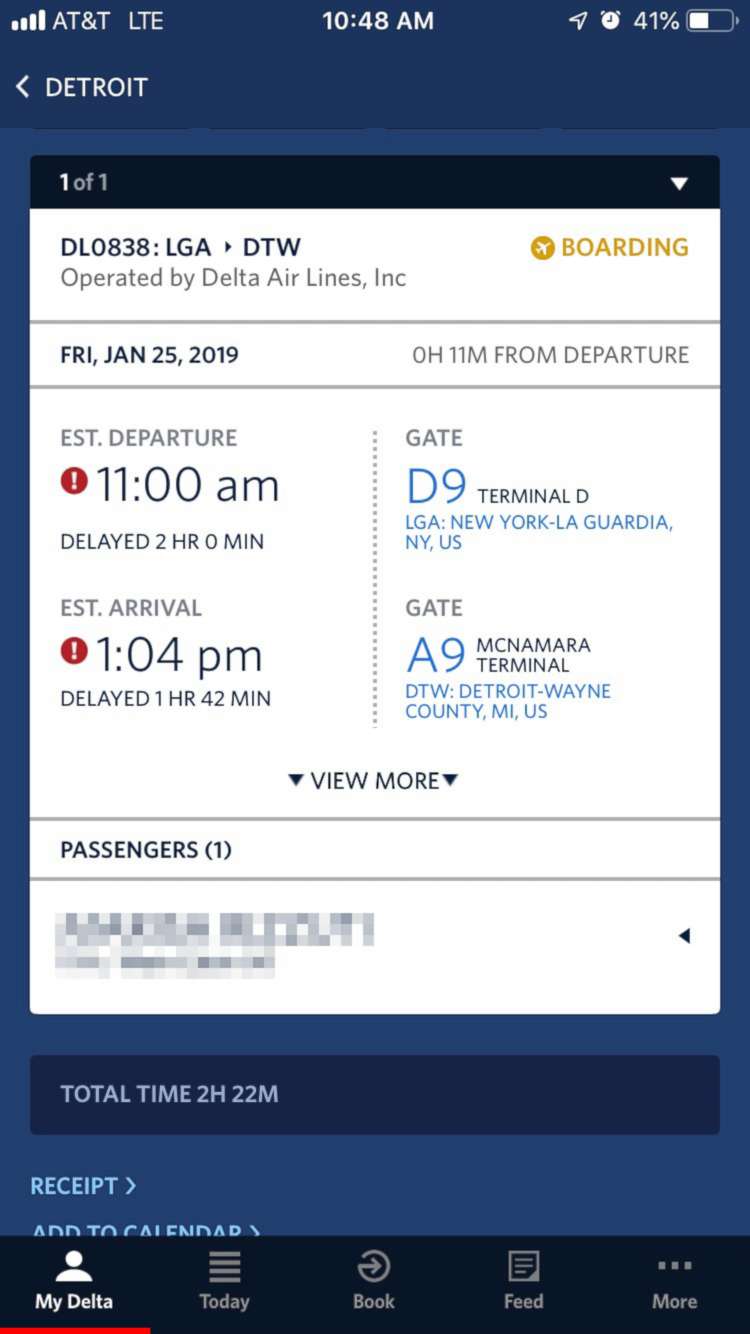The screenshot on the cell phone displays a detailed view of a travel itinerary. Starting from the top, the header background is navy blue, featuring indicators for cell phone signal strength bars, the carrier name "AT&T," and the network type "LTE." In the center, the time is displayed as 10:48 AM, next to indicators showing an active alarm and a battery level at 41%, with the battery icon filled in white.

Below this header, there is a left arrow followed by the text "DETROIT" in capital letters. The next section has a lighter blue background transitioning into a black area that serves as a heading, reading "Banner." To the right of this heading, it indicates "1 of 1" accompanied by a downward arrow key.

The screenshot then details a travel itinerary in a white print background with black text. It lists the flight number "DL0838" with the route "LGA-DTW," noting that the flight is operated by Delta Airlines, Inc. The status "Boarding" is highlighted in gold. Further information includes:

- Flight date: Friday, January 25, 2019
- Estimated departure time
- Estimated arrival time
- Gate number for departure
- Gate number for arrival
- Option to view more details
- Passenger information
- Total flight duration: 2 hours and 22 minutes

At the bottom, the interface label "My Delta Today" and a book feed option are visible.